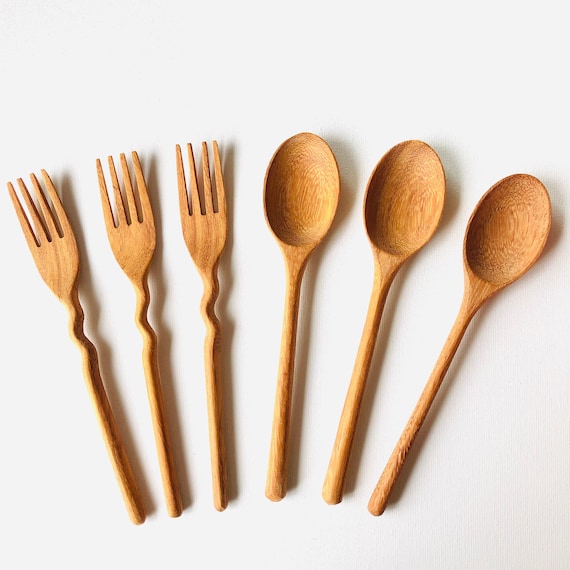This square photograph features a meticulously arranged set of six handcrafted wooden utensils on a pristine white background. To the left side, there are three uniquely designed forks, each with four tines and a distinctively curved transition at the base of the handle, which then straightens out towards the end. To the right, there are three wooden spoons, characterized by a large, slightly flattened oval scoop and a slim handle that widens towards the end. The utensils are fanned out, with their handles closer together at the bottom, creating an artful display. Soft shadows beneath each piece hint at a light source positioned above, highlighting the intricate details and smooth, light-colored wood finish.